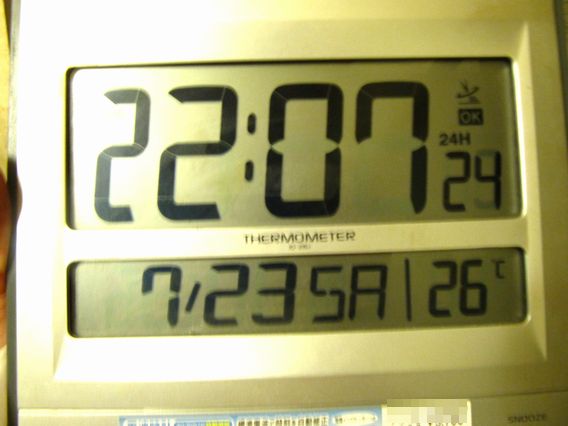This is a detailed close-up photograph of a rectangular thermostat, tinted yellow due to the lighting. The thermostat features two distinct display areas. The top display shows '2207' with '24H' in small print next to it, followed by the number '24' beneath. Below this display, the word 'Thermometer' is engraved on the plate. Further down, a smaller digital screen displays '7/235A'. A dividing line separates this from the reading '26°C'.